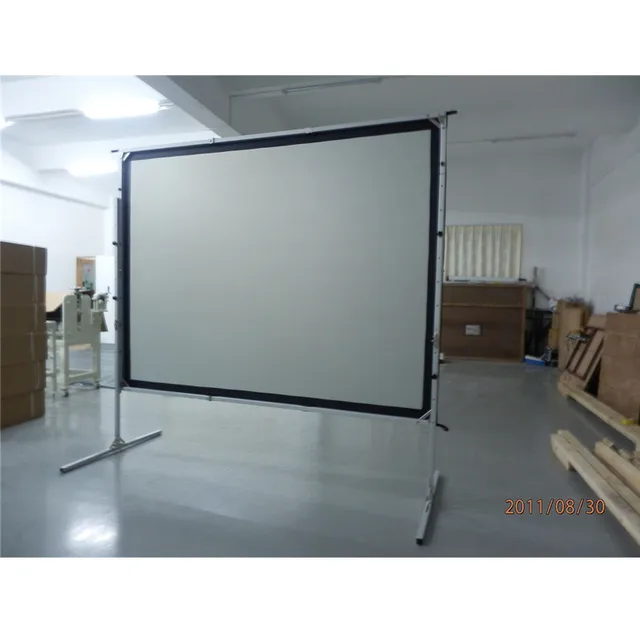In a spacious room with white walls and ceiling, illuminated by bright lights concentrated on the left side, stands a large, square whiteboard at the center. The whiteboard, bordered by a black rectangular frame, is supported by two sturdy, silver metallic legs. The floor beneath is green. On the left side of the floor, there's a stack of cardboard boxes and a white wooden chair resting next to them. To the right, various wooden materials, including wooden knocks lying on the ground and wooden plates leaning against the wall, can be observed. At the back of the room, a dark brown cabinet stands against the wall with a heater situated above it. The time stamp, dated August 30, 2011, in bright orange, is located at the bottom right-hand corner of the image.